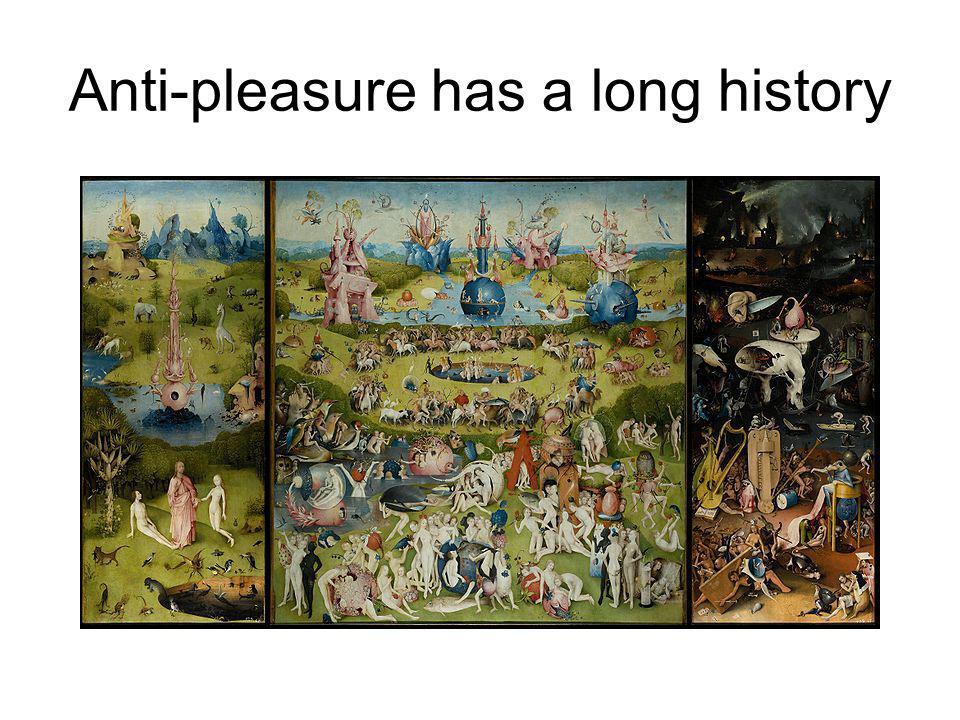This detailed vintage painting, titled "Anti-Pleasure Has a Long History," is presented in a large, long frame divided into three distinct panels, each encapsulating a different scene. The caption in black letters atop the image reads, "Anti-Pleasure Has a Long History."

The left panel depicts a surreal landscape with blue mountains and green fields in the background. In the foreground, three half-dressed individuals engage in conversation with a figure in a pink robe. Various fantastical animals, unlike any seen before, populate the scene, adding to the magical atmosphere.

The central panel is brimming with activity and features numerous naked or semi-naked figures amidst a sunny or partially cloudy setting. The scene resembles an old-worldly festival where people indulge in various pleasures and sufferings. Outlandish structures, including spheres with towers emerging from them, add to the chaotic yet fascinating tableau, with the backdrop hinting at water bodies.

The right panel contrasts sharply with the others, dominated by dark and muted colors like blacks and browns. The background showcases dark castles and buildings under a nighttime sky. The foreground is filled with grotesque demonic creatures and fragmented body parts, with people appearing to be in different stages of torment and torture.

Overall, the painting combines elements of fantasy, historical reference, and abstract imagery to convey a compelling narrative about human pleasure and suffering throughout history.